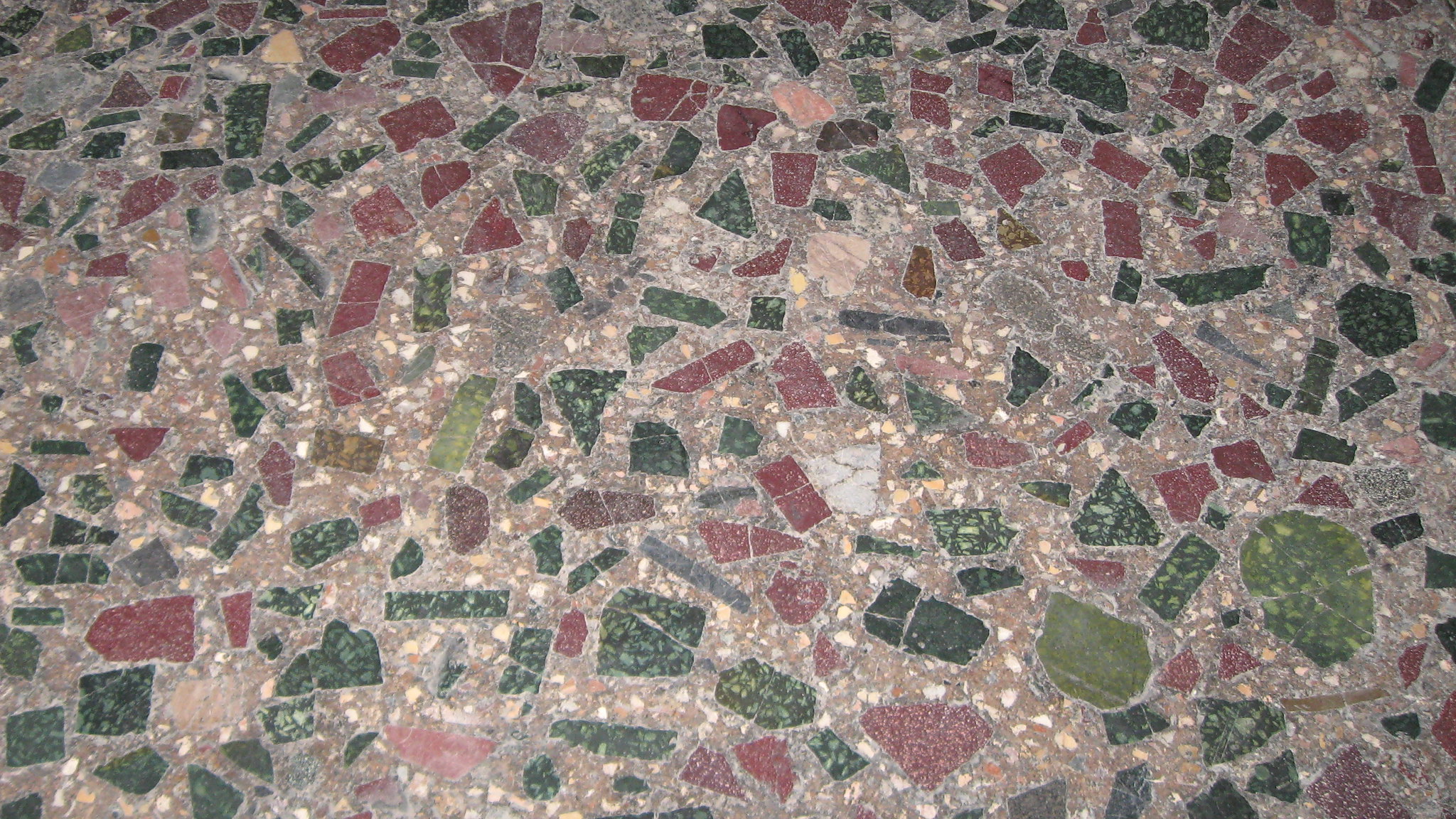This photograph showcases a richly textured, mosaic-like floor composed of irregularly shaped and sized tiles. The primary material appears to be a pinkish-brown cement that serves as a binding matrix for the scattered stones. Dominating the design are dark green and dark crimson (maroonish) tiles, with shades ranging from moss to forest green for the green tiles. Smaller, beige or cream-colored stones are interspersed throughout, adding a contrasting texture and color that enhances the pattern. The surface, possibly rough to the touch and indicative of age and significant foot traffic, suggests an important, well-worn pathway or a utilitarian surface like a countertop. Despite its somewhat worn and chaotic appearance, the floor seems to have been meticulously arranged to create an intricate, multicolored mosaic that is visually striking.